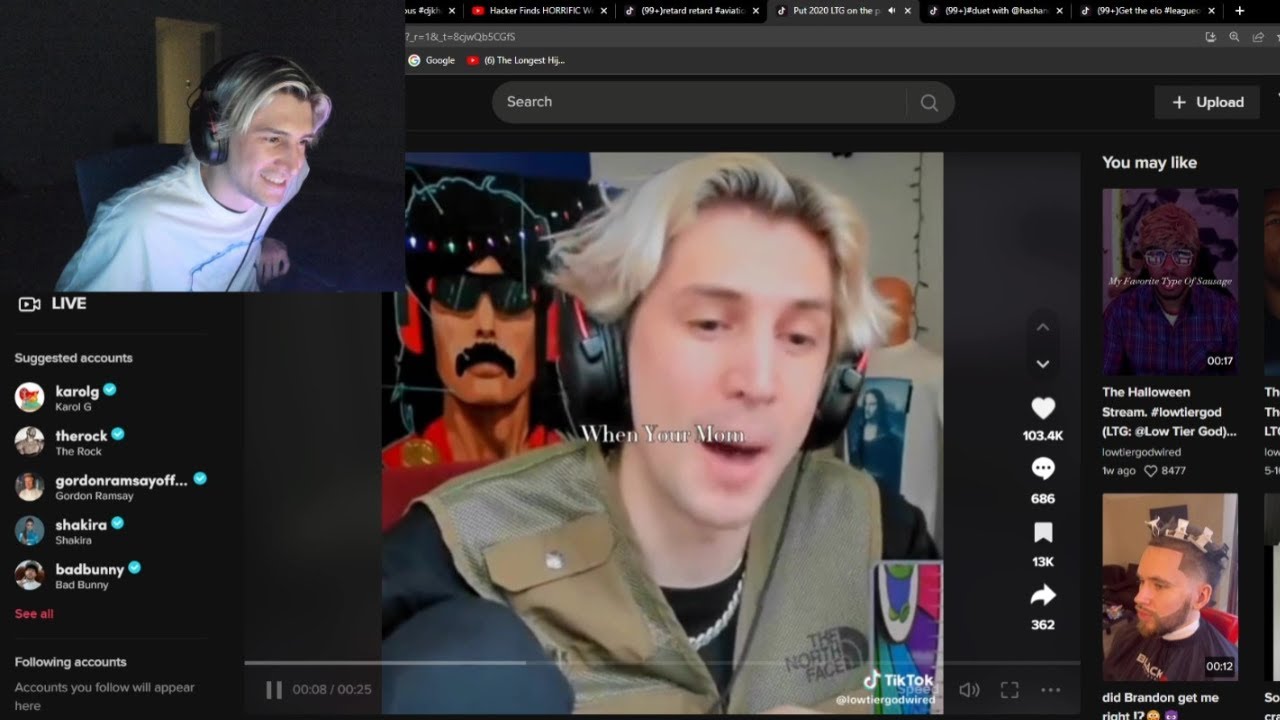The image is a detailed screenshot of a YouTube browser page. In the top left corner, there's a square video box featuring a man in a white shirt wearing a headset, looking down or towards the right side of the page. Adjacent to this, the main YouTube interface is visible.

In the middle of the screen, a TikTok video is playing, signified by the TikTok logo in the bottom right corner. White text overlaying the video reads "win your mom," and the video appears to show the same man, the one seen in the smaller video box, watching content he previously uploaded to YouTube.

At the bottom left of the screen, the "Suggested accounts" section displays various accounts, each marked with blue check marks denoting their verified status.

On the right side of the TikTok video, there is a column of icons arranged vertically, each with corresponding interaction metrics. At the top is a heart icon indicating 103.4 thousand likes, followed by a chat bubble icon with 686 comments. Below that is a bookmark icon showing 13,000 bookmarks, and lastly, an arrow icon pointing left, which indicates 362 shares.